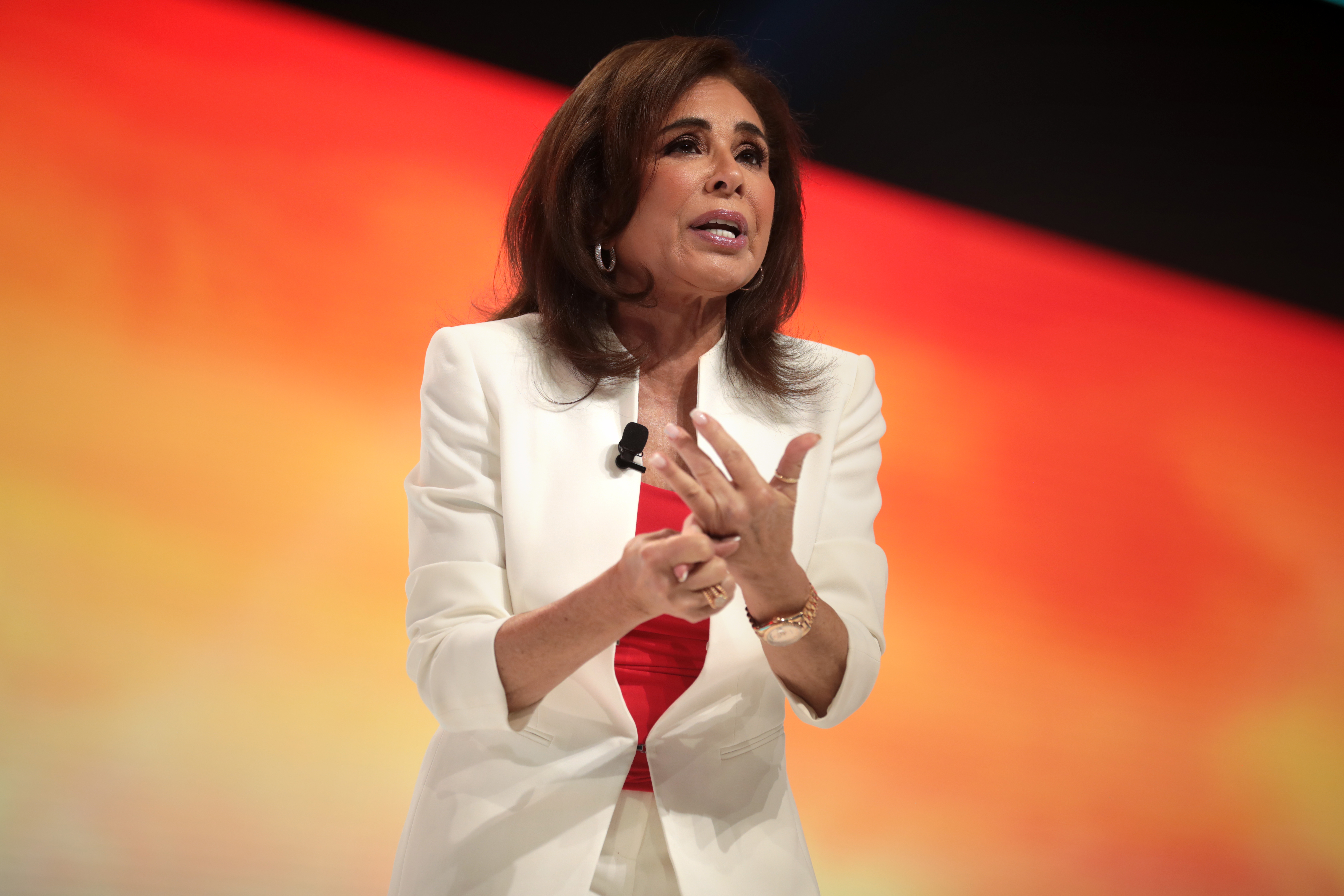The image features an older, well-dressed woman, likely in her 50s or 60s, giving a talk. She is wearing a white suit with a three-quarter sleeve jacket and white pants, complemented by a vibrant red shirt underneath. Her hazel-brown, shoulder-length hair frames her face, which is adorned with pink lipstick and subtle makeup. She has silver earrings, rings on her well-manicured fingers, and a gold wristwatch on her left hand. A small microphone is clipped to the lapel of her jacket. She is gesturing with her right hand, enumerating by holding down one finger, as she speaks. The background is blurred with an orange and black gradient, resembling a planetary or sunrise effect, which adds an intriguing, almost celestial backdrop to her presentation.